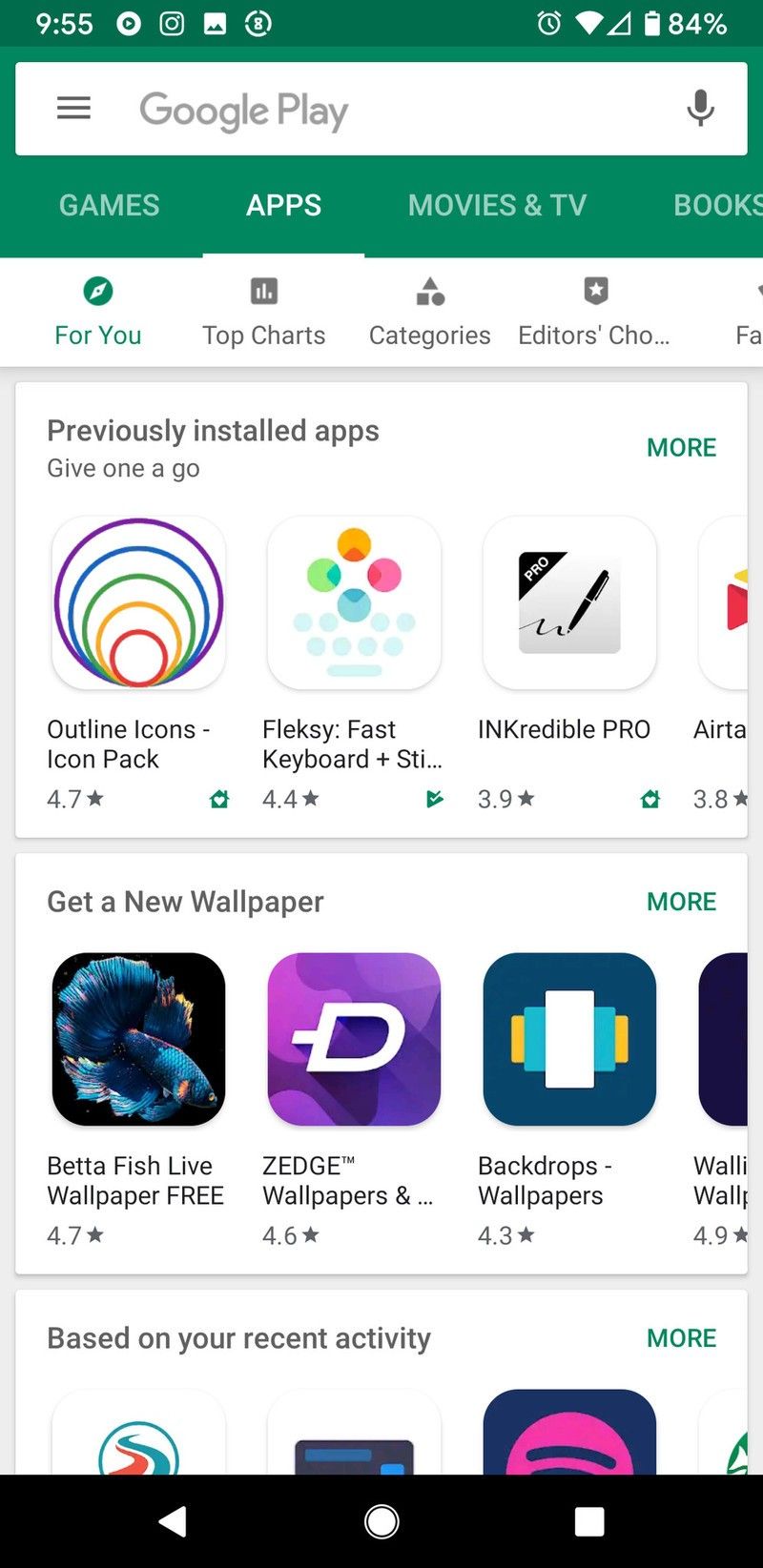The image showcases the layout of a webpage, likely from the Google Play store, with distinct sections and a detailed top banner. 

At the very top, there's a dark green banner featuring a lighter colored text, either white or light green, displaying the current time on the top left as "9:55". Adjacent to the time, a series of symbols are spread across towards the middle, with icons resembling a clock and a battery indicator showing "84%" on the top right.

Beneath the green banner, a white banner highlights "Google Play". Directly below, the green banner showcases navigation tabs including "Games", "Apps", "Movies & TV", and "Books" arranged from left to right.

Continuing downwards, another white banner has several options such as "For You", "Top Charts", "More Categories", and "Editor's Choice". The "For You" section is highlighted in green. Towards the far right, an incomplete label "FA" is visible, partially off the page.

Under the "For You" section, previously installed apps are listed with a prompt "Give One a Go". The listings feature outline icons on the left with a variety of colored circles within a circle. Moving right, a category labeled "FlexKey" alongside other small circles appears, followed by "Incredible Pro" with some intricate design elements.

Further down, there's a prompt to "Get a New Wallpaper", showing "Betta Fish Live" on a black background with colorful fish. Below are various designs with labels underneath each.

At the very bottom of the visible area, there's a segment titled "Based on Your Recent Activity" showcasing different items, though partially cut off at the bottom of the page.

Finally, a black bar is seen at the bottom featuring navigation elements: an arrow pointing left on the left side, a circle in the middle, and a white bar on the far right.